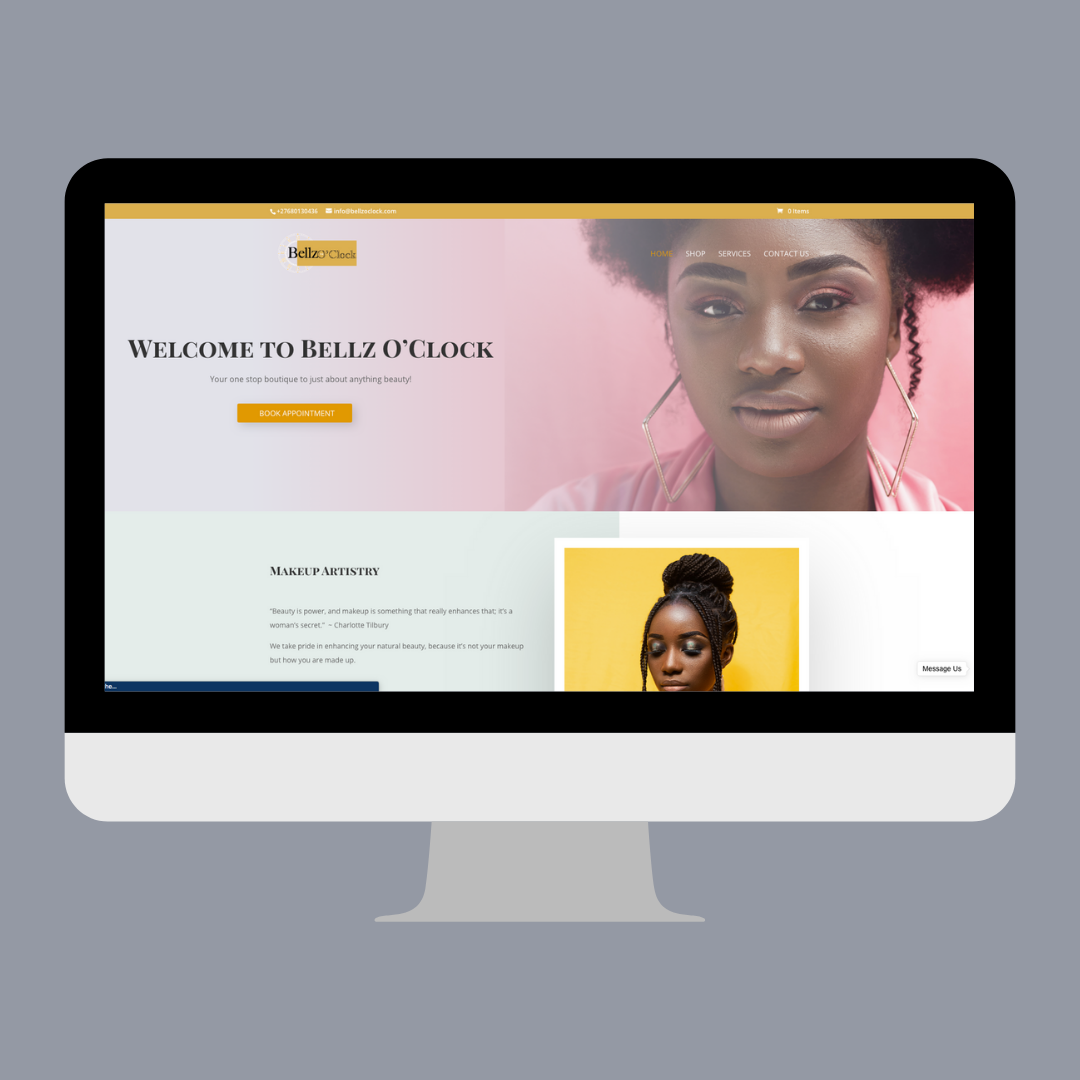The image features a desktop computer displaying a website. Positioned just slightly off-center to the left at the top of the screen, the title "Bells O'Clock" is prominently displayed, with "Bells" intentionally spelled with a "Z" at the end. To the right of this title is a close-up photo of a woman. On the left-hand side below the title, there is a welcoming message that reads, "Welcome to Bells O'Clock." Directly beneath this introductory note, a tagline states, "Your one-stop boutique for just about anything beauty." Below this, there is a yellow-orange box with text that reads "Book Appointment." Additional smaller descriptions are seen scattered below the box, further detailing the website's offerings.